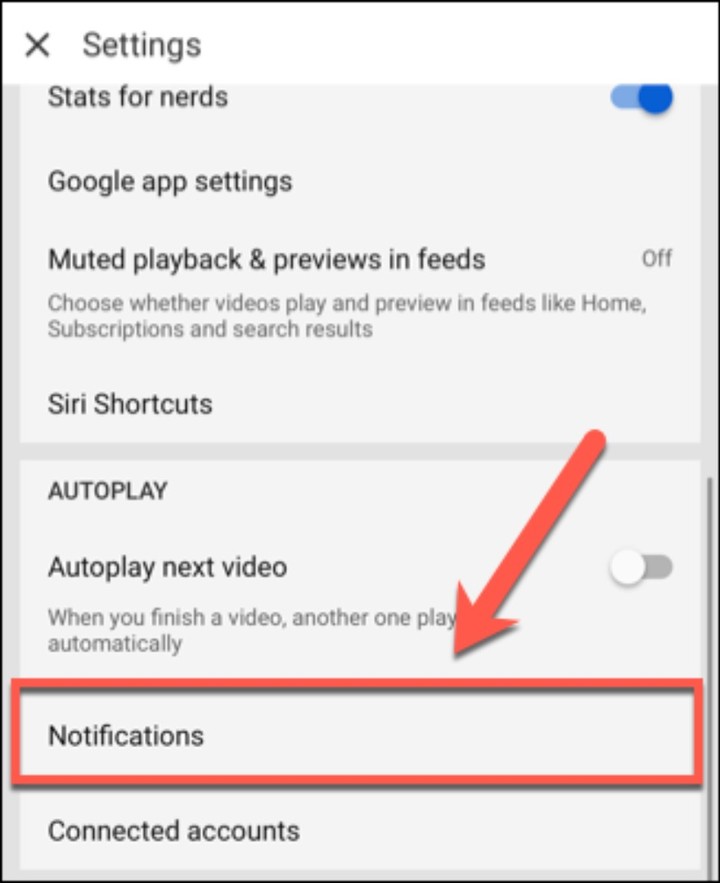### Detailed Descriptive Caption:

The image is a screen capture of a settings menu from what appears to be a web or mobile application, highlighted for instructional purposes. The focal point is a section labeled "Notifications," clearly demarcated with a red bar and pointed to by a red arrow, indicating its relevance in the context of the guide. Within the broader settings menu, several options are visibly configured:

1. **Stats for Nerds**: A quirky feature toggled 'on' with a slider, likely providing advanced metrics or diagnostics to users interested in technical details.
2. **Google App Settings**: This section contains various preferences related to sync and integration with Google services.
3. **Muted Playback & Preview in Feeds**: This option is toggled 'off.' It includes a descriptive note explaining that enabling it would result in videos playing silently and previewing across different feeds such as Home, Subscriptions, and Search Results.
4. **Siri Shortcuts**: Another tab option possibly suggesting voice command configurations with Siri, Apple's virtual assistant.
5. **Autoplay**:
   - **Autoplay Next Video**: This functionality, currently turned 'off,' manages whether a next video in sequence starts playing automatically.

Below the highlighted "Notifications" area, there's another section titled "Connected Accounts," hinting at options for managing linked social media or service accounts.

This image, marked with clear visual indicators, seems to be intended for educational or training material, guiding users on how to navigate and manage their app settings effectively.